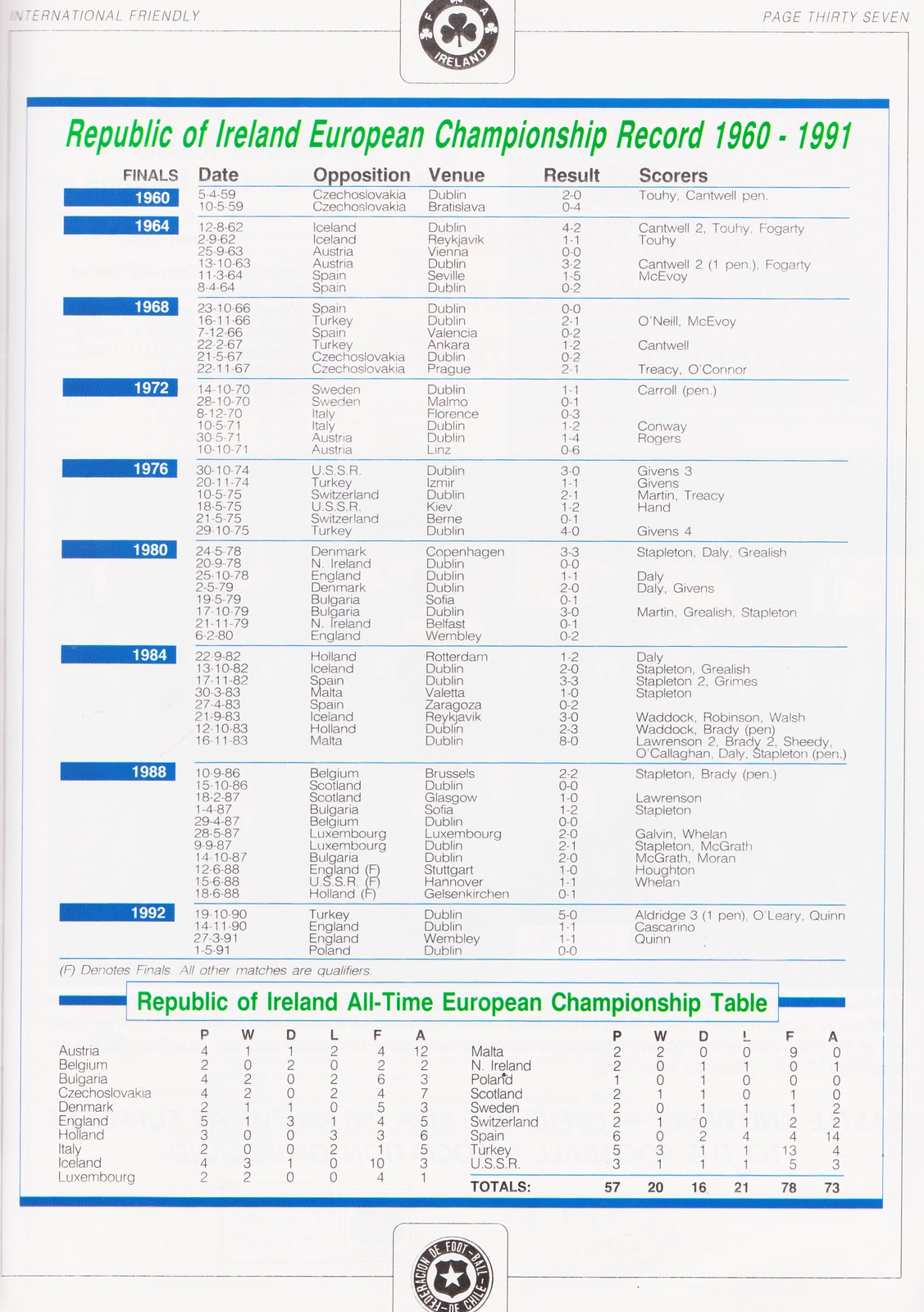The image is a detailed scorecard for the Republic of Ireland's European Championship records from 1960 to 1991, displayed on a white background. In green letters at the top, it reads "Republic of Ireland European Championship Record, 1960 to 1991." Below this heading is an insignia featuring a shamrock. The left side lists the dates of the finals, ranging from 1960 through to 1992 (yet to be completed), each year highlighted in blue boxes with white text. Next to these dates, columns are labeled for the date, opposition, venue, result, and scorers, all neatly organized. At the bottom of the page, another green text reads "Republic of Ireland All-Time European Championship Table," listing countries with their scoring records. Dark blue borders frame the top and bottom of the page. Additionally, a symbol with a star and indistinguishable writing appears at the very bottom. The format ensures easy readability and a clear breakdown of information by year.